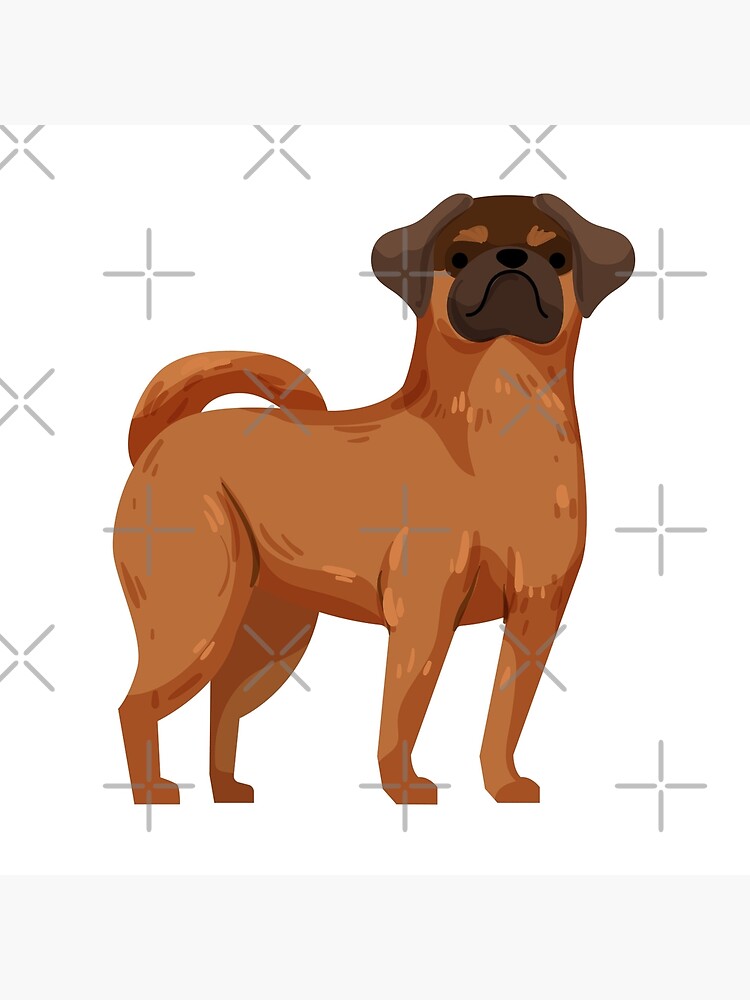This image is a perfectly square, digitally created animation of a cartoonish dog set against a white background sprinkled with semi-transparent gray Xs and plus signs arranged in an evenly spaced pattern. The dog is centrally positioned, facing directly towards the viewer. Its compact and stout body is predominantly a light tan brown, adorned with lighter tan pops, while its head, ears, and snout exhibit a deeper shade of brown. The dog’s facial features include simple brown dots for eyes and nose, and an upside-down "U" shape for the mouth. Its long tail curves gracefully upwards to touch the center of its back. There are no additional elements such as other dogs, people, text, or artist signatures in the image, drawing full attention to the stylized, vector-like illustration of the solitary dog.